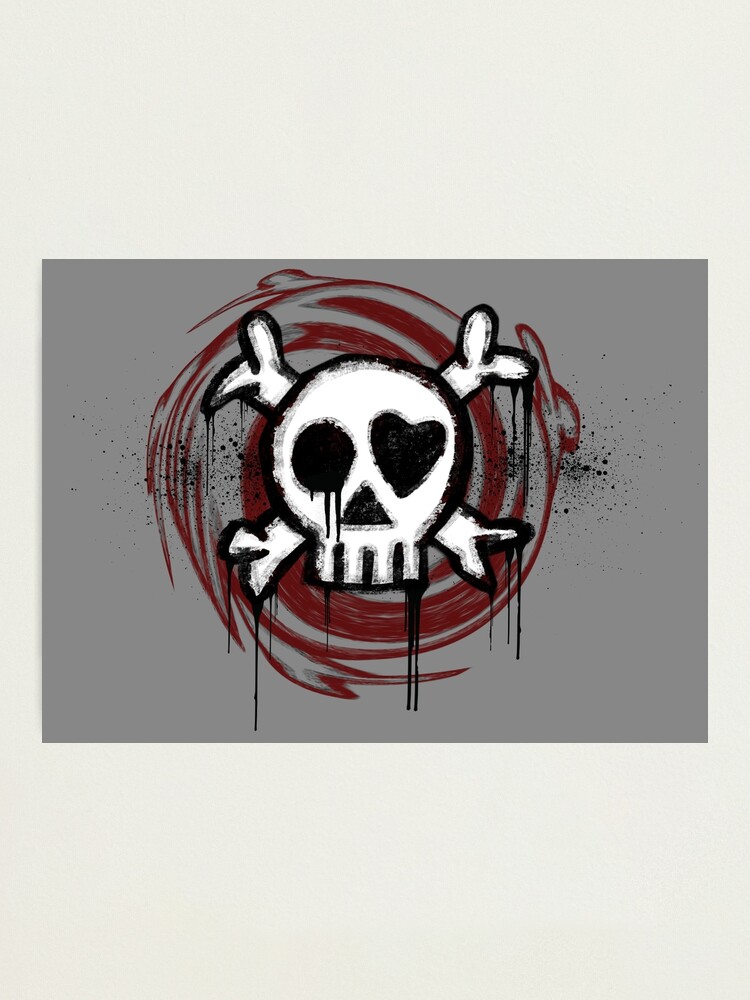The image is a horizontal rectangle with a gray background, featuring a digitally repainted artwork. At the center, a white skull and crossbones symbol is prominently displayed, reminiscent of the common danger symbol for chemical pesticides. The skull's left eye socket is distinctly heart-shaped, while the right eye socket is a perfectly round circle. Both eye sockets and the nose, which is a perfect black-filled triangle, stand out sharply against the white skull. Surrounding the skull and crossbones is a jagged, maroon swirl pattern, forming a clockwise spiral reminiscent of a snail's shell. Speckles of black paint are scattered across the image, giving it a textured appearance. The skull and crossbones are further outlined with a dripping black border, enhancing the graphic, almost hand-painted aesthetic of the artwork.